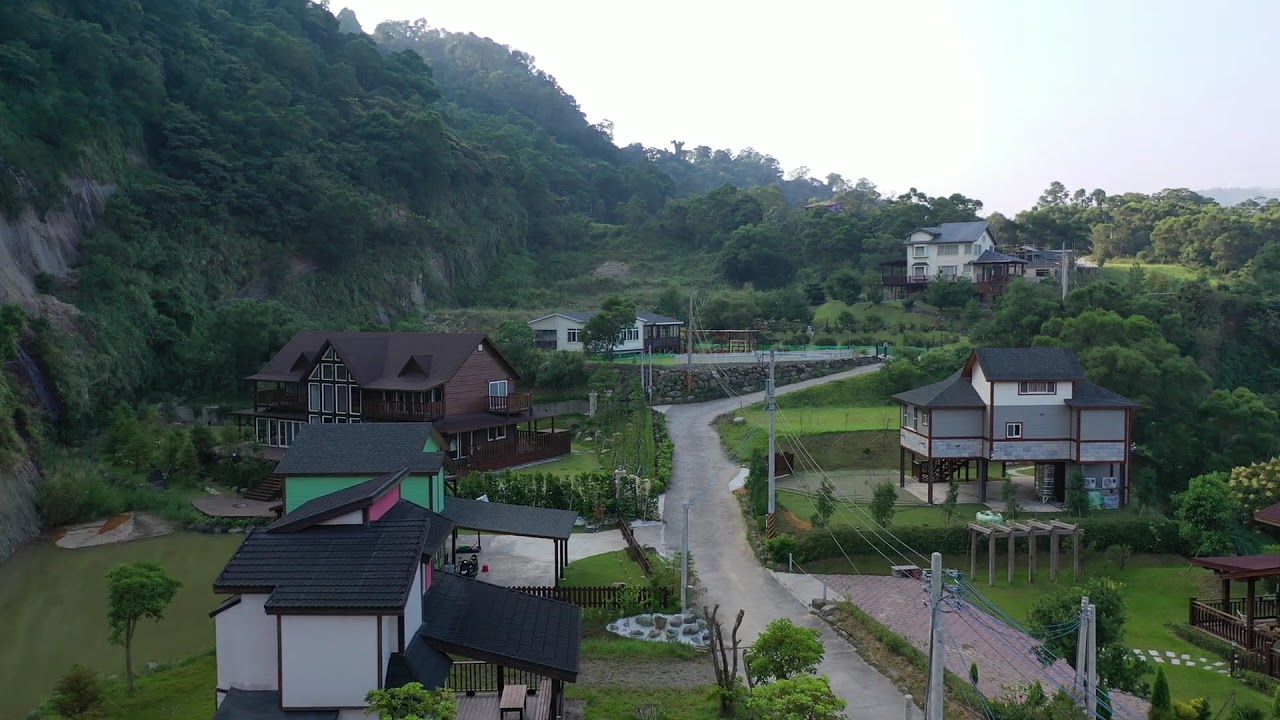This aerial color photograph, taken with a drone and in landscape orientation, depicts a secluded neighborhood at the foothills of a mountainous region. The scene is reminiscent of a European village, featuring six or seven distinct dwellings in a variety of colors, predominantly gray with dark roofs but also including a notable white house with a black roof and a partly visible lime green house. These homes range from two to four stories high and are nestled amidst well-manicured green grass, bushes, hedges, and an abundance of tall, dark green trees. A windy grey road meanders through the center of the village, creating a picturesque divide between the houses. In the background on the upper left, large hills and mountains rise up, thickly covered in lush, verdant trees, enhancing the serene and rustic charm of this mountaintop enclave.